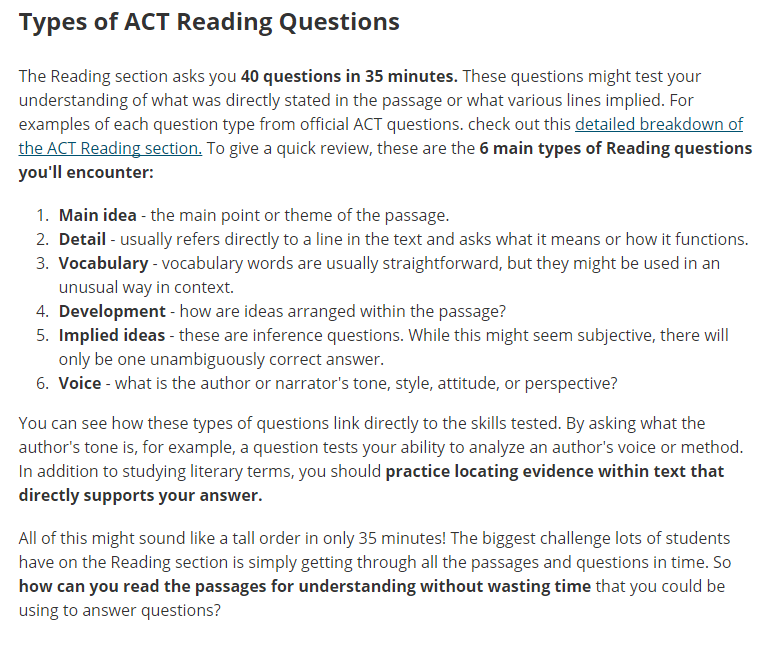**Caption:**

The image features a white background filled with text, all pertaining to the types of questions found in the ACT Reading section. The main heading, "Types of ACT Reading Questions," is prominently displayed at the top. Below the heading, an introductory paragraph highlights that the ACT Reading section consists of 40 questions to be answered in 35 minutes. These questions assess both direct and implied comprehension of the passage content. For those looking to delve deeper, the text encourages reviewing a detailed breakdown of the ACT Reading section, with this phrase being underlined for emphasis.

Following the introduction, the text lists six main types of reading questions commonly encountered on the ACT:

1. **Main Idea**: Questions about the primary point or theme of the passage.
2. **Detail**: These questions reference specific lines in the text, asking about their meaning or function.
3. **Vocabulary**: Focused on understanding vocabulary words, sometimes used in unusual contexts.
4. **Development**: Concerned with how ideas are structured within the passage.
5. **Implied Ideas**: These inference questions require identifying the only unambiguously correct answer.
6. **Voice**: Analyzes the author or narrator's tone, style, attitude, or perspective.

The text further explains how each question type is designed to test specific skills, such as analyzing an author's voice or method. It emphasizes the importance of studying literary terms and practicing the identification of textual evidence to support answers. Lastly, it acknowledges the common challenge of managing time effectively while reading and answering questions, and prompts readers to consider strategies for efficient reading comprehension.